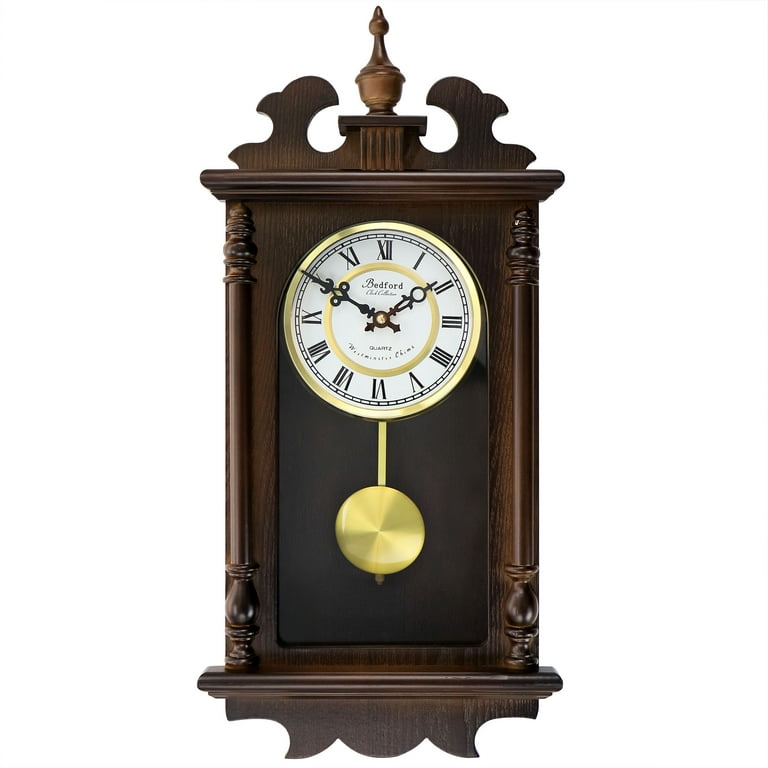This is a detailed close-up photograph of a vintage-style, dark walnut wall clock, crafted to resemble a smaller version of a grandfather clock. The clock, likely around 20-21 inches tall, features a rectangular wooden body with intricate dark brown woodwork. The design includes a ledge on the front and decorative borders at both the top and bottom. The clock face, accented with a gold trim, is round with a white center, showcasing black Roman numerals and two intricately designed black hands indicating the time near 10:02. Below the clock face, a gold pendulum hangs gracefully. Flanking the clock face are two ornate pillars, adding to its classic aesthetic. The clock, from the Bedford Clock Company, also features an arched piece of glass in the middle and a striking golden second hand that swings below the face.